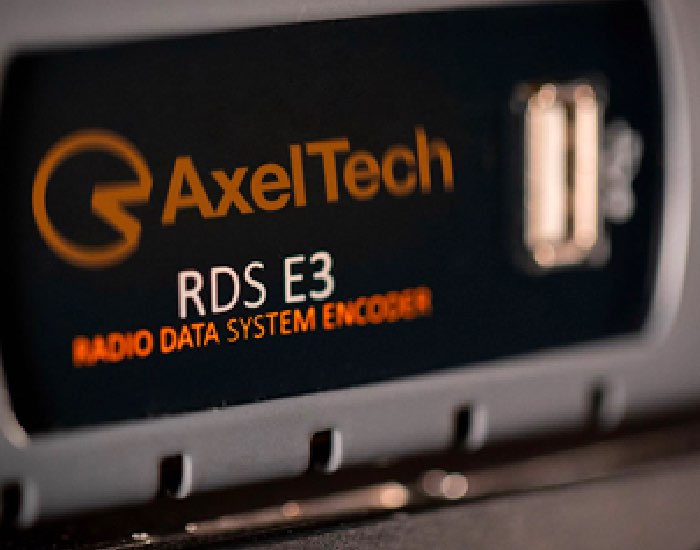This image features a close-up of an electronic device, specifically a Radio Data System Encoder, identified by the model name RDS-E3. The central rectangular gadget has a black front panel with silver or gray background edges. Dominating the top section of the black front is the brand name "AxelTech" in bold orange letters, accompanied by a distinctive Pac-Man-like logo. Directly below this in white text is the model identifier "RDS-E3", and further down, in slightly blurry but discernible orange writing, is the label "Radio Data System Encoder." A vertical USB slot is positioned to the right on the front panel, emphasizing the functional aspect of the device. The detailed mixture of colors—black, silver, gray, and orange—adds to the visual interest of this technology-focused product image.